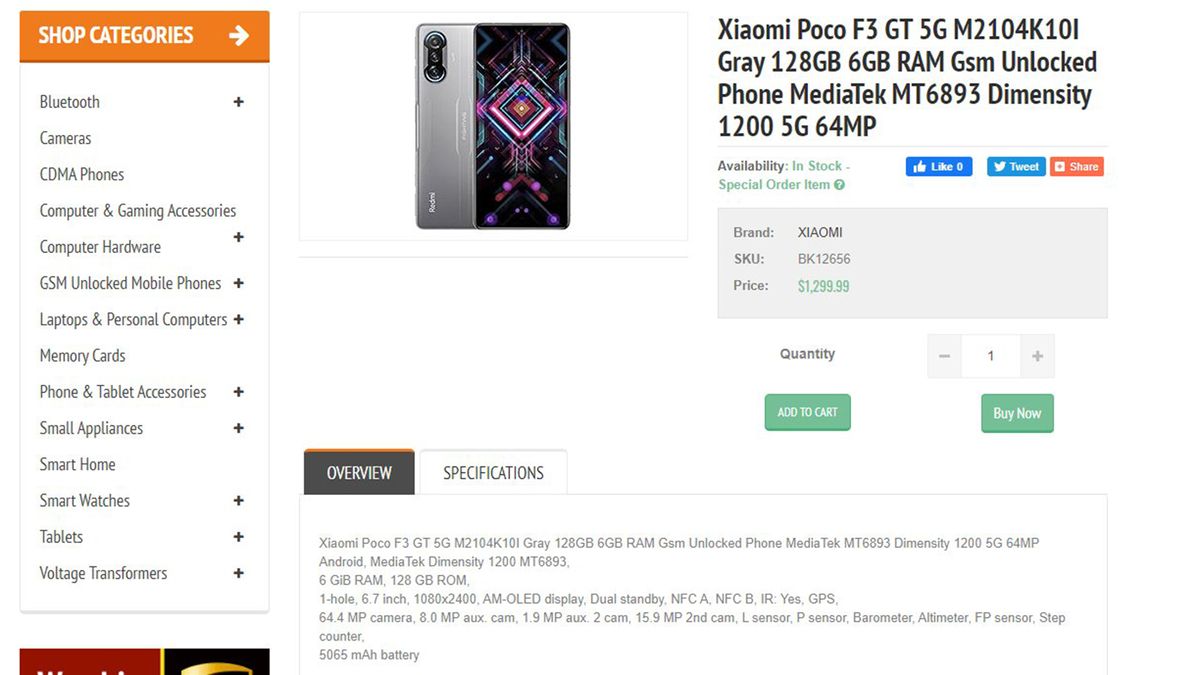This image depicts a section of an e-commerce webpage showcasing a product listing for a phone. 

On the left side of the page, an orange header with white text reads "Shop Categories" and features an arrow pointing to the right. Below this heading, a list of categories is displayed on a white background with black text. Each category name is accompanied by a plus sign on the right side. The categories listed are:
- Bluetooth 
- Cameras
- CDMA Phones
- Computer and Gaming Accessories
- Computer Hardware
- GSM Unlocked Mobile Phones
- Laptops and Personal Computers
- Memory Cards
- Phone and Tablet Accessories
- Small Appliances
- Smart Home
- Smart Watches
- Tablets
- Voltage Transformers

Moving to the main section of the page, a featured product—a phone—is highlighted. The left side of this section displays half of the phone, showing both the front and back. The back of the phone features a vertical camera array with three lenses stacked on top of each other, and the phone case is a shiny dark gray. The front of the phone showcases a design with geometric shapes. The product is identified as a "XIA-OMI Poco F3 GT 5G" with a gray color and 528 GB of storage. The product is noted to be in stock and categorized as a special order item.

To the right of the product image, users have the options to like, tweet, or share the product. The page provides additional details including the brand, SKU number, and price, which is prominently displayed in green text as $1,299.99. 

Below the price, the quantity selection is presented with a number 1 displayed in a box. Adjacent to this are two green buttons with white text, labeled “Add to Cart” and “Buy Now.” 

Further down, an overview of the product is visible, alongside a specifications section. The overview box has an orange line at the top and is filled with a dark gray color, featuring white text, while the specifications box is aligned to its right.